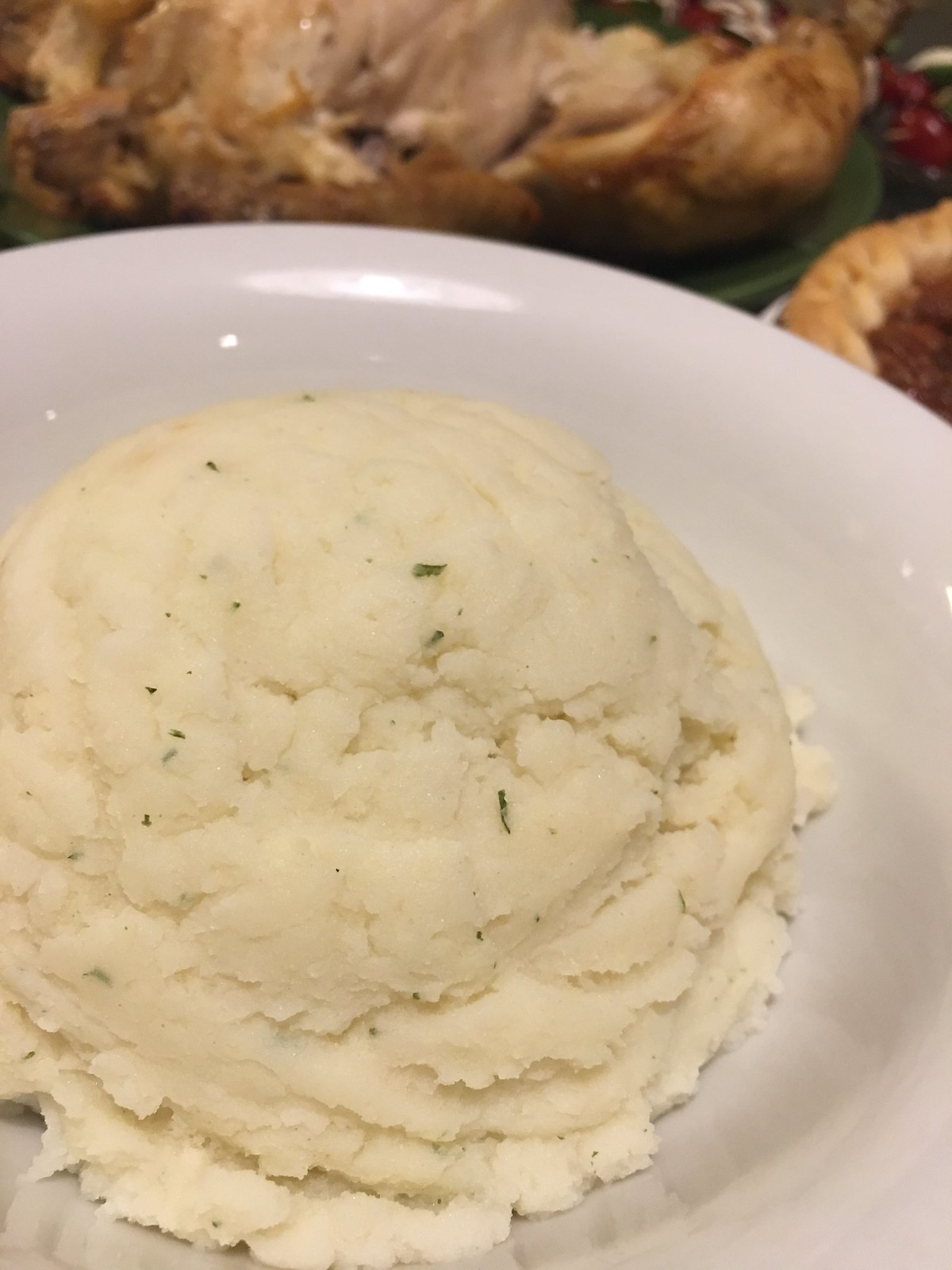In this detailed image, we see a close-up of a large, rounded scoop of mashed potatoes, resembling the shape of an ice cream scoop, sitting on a white ceramic plate. The mashed potatoes have a slightly off-white or yellowish tint and are speckled with green herbs, possibly chives or parsley, adding a hint of texture and color. The white ceramic plate occupies the majority of the image, reflecting light to emphasize the creamy texture of the potatoes. 

In the background, partially blurred, there is a green plate featuring what appears to be carved roasted turkey, displaying a mix of brown and tan hues. To the upper right, the crust of a dessert, likely a pecan pie, is visible with its brown filling and tan crust. The background elements provide a rich, warm contrast, making the mashed potatoes on the white plate the focal point of this cozy kitchen or dinner table scene.